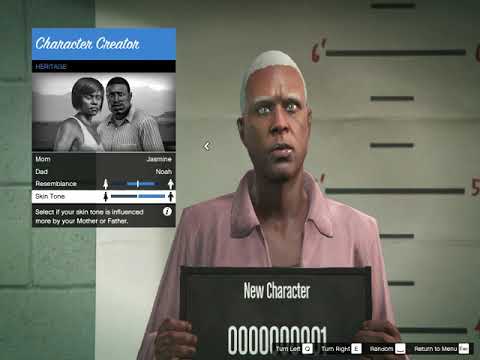This image resembles a mug shot from a video game. The individual pictured is holding a board typically used in mug shots, which displays the text "New Character" and the identification number "0000000000001." The person is wearing a pinkish shirt and has short greyish-white hair. The background features a height chart on the wall, with the 6-foot mark visible just above the person’s left shoulder, on the right side of the image. The man is directly facing the camera. On the left side of the image, there is a character creation interface where a male and female character are standing chest to chest, both facing the camera.